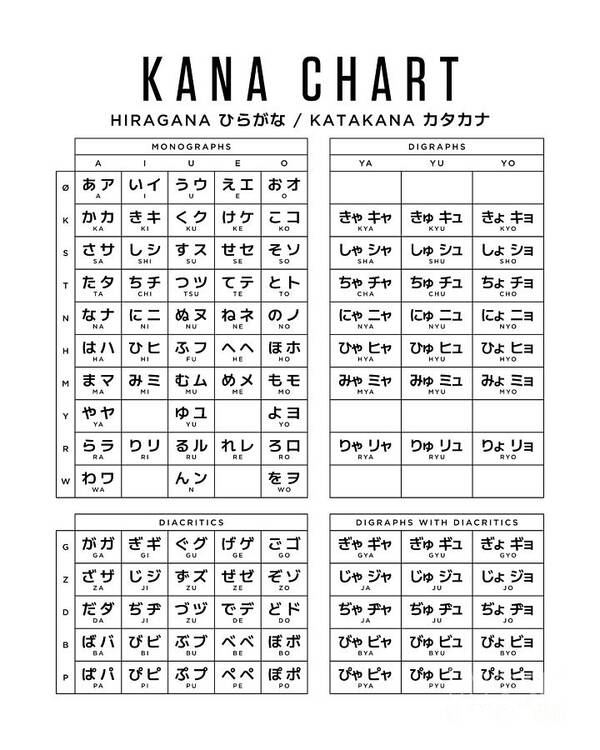This image features a comprehensive Kana Chart presented in black and white, showcasing a detailed comparison of Japanese kana characters and their English counterparts. The chart is segmented into four distinct sections, each meticulously labeled at the top. The first section, "Monographs," displays individual kana characters alongside their corresponding English transliterations. The second section, "Digraphs," illustrates combined kana characters and their English equivalents. The third segment is titled "Diacritics," presenting kana characters modified by diacritical marks, thereby altering their pronunciation. The final section, "Digraphs with Diacritics," merges these concepts to show kana digraphs with additional diacritical modifications. Arranged along the axes of the chart, you can find the English vowels A, I, U, E, O, and various consonants including K, S, T, N, H, M, Y, R, and W, guiding viewers through the intricate relationships between Japanese kana and English sounds.